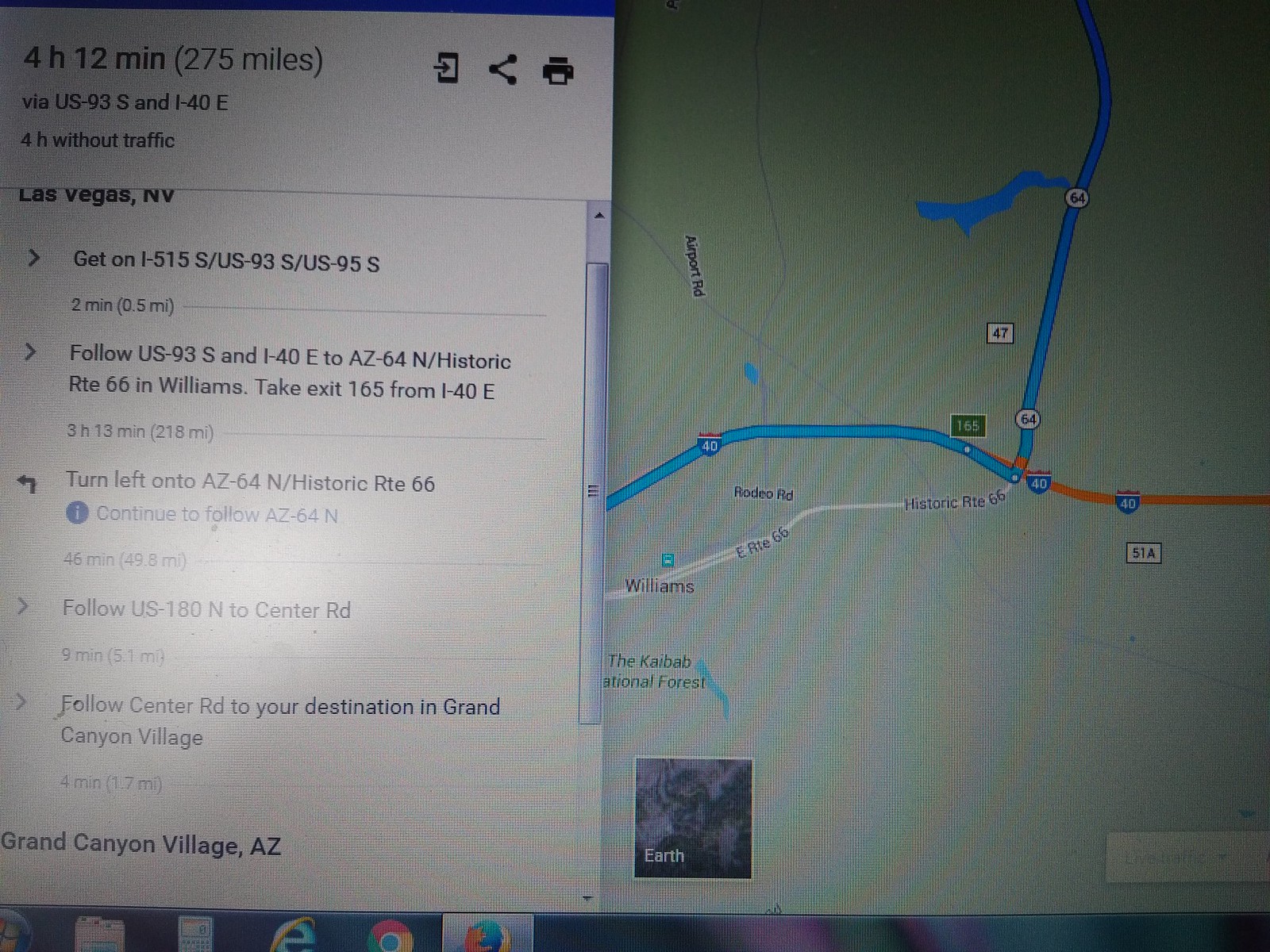The image displays a computer monitor with the screen turned on. On the left side of the screen, there is a map with directions. The background of the map is white, with blue and black text detailing a route that takes 4 hours and 12 minutes, covering 275 miles to reach Canyon Village, Arizona. The directions begin with "Get on I-515 South US-93" and continue along US-93. At the bottom of the screen, it specifies the starting point as Las Vegas, Nevada, with the destination being Canyon Village, Arizona.

In the interface of the screen, several browser icons are visible at the bottom, including the blue Internet Explorer logo from Microsoft, the Chrome logo represented by a circle with shades of green, orange, and yellow, and the Firefox logo for that browser. On the right side of the screen, detailed map markings illustrate the route to the destination, providing a clear visual guide for the journey.